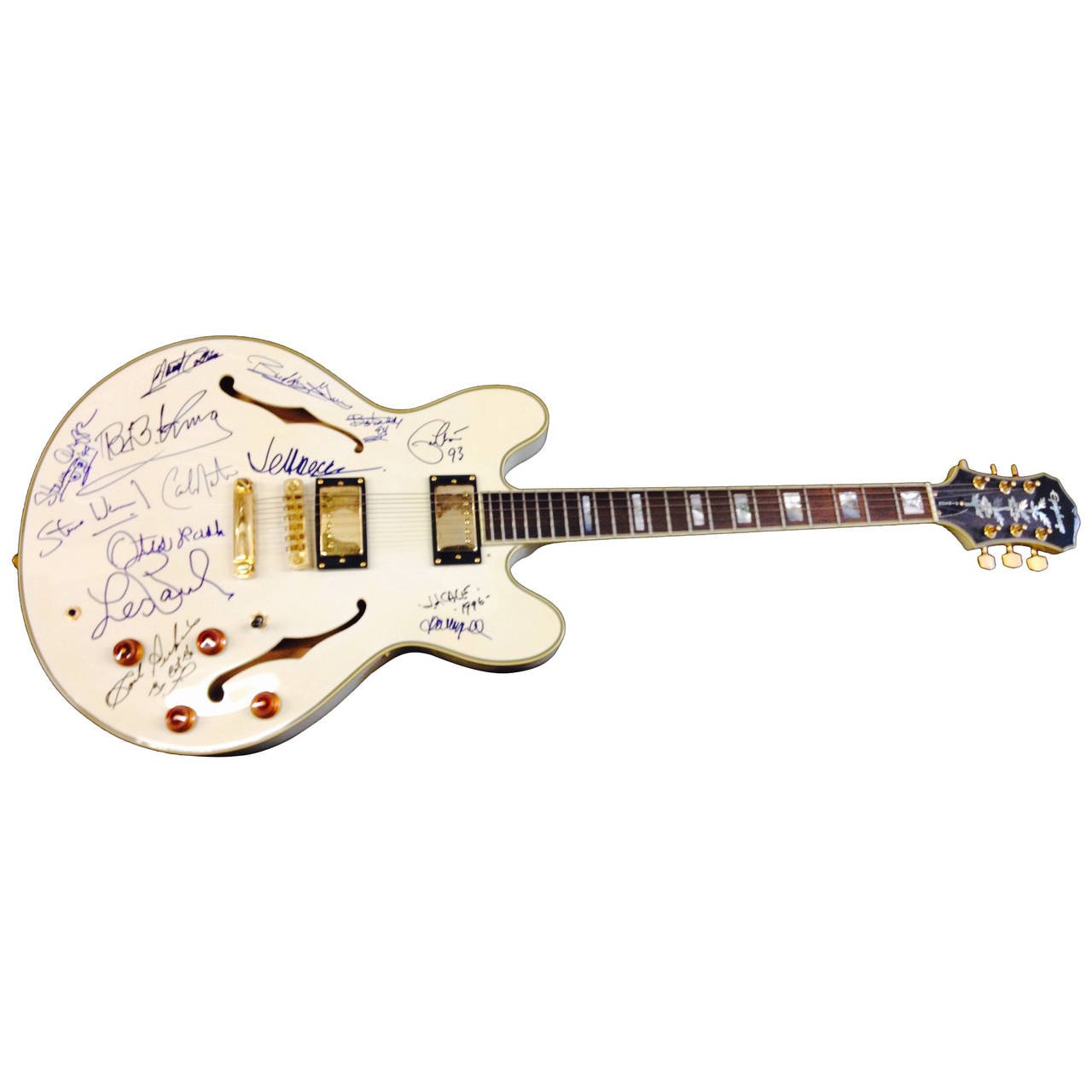This photograph showcases a stunning white Epiphone Casino electric guitar, positioned horizontally against a white backdrop. The body of the guitar is cream and white, resembling the kind often played by John Lennon. The dark brown neck features black at the headstock, which proudly displays the Epiphone logo with gold tuner knobs. The guitar is adorned with a variety of signatures from renowned musicians, including prominent ones from BB King and Les Paul near the middle, and Otis Redding centrally. The guitar also boasts elegant details like gold pickups, bronze-colored knobs, a pickup selector, a gold tailpiece, and hardware with pearl block inlays. The signatures, some clearly legible and others more obscure, attest to its historical and musical significance, making it a visually and culturally captivating piece.